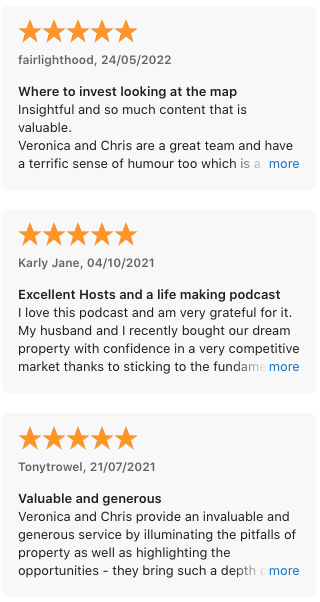A screenshot showcasing three five-star customer reviews highlights outstanding praise for a particular podcast. The most recent review, dated May 24, 2022, is by Fair Lighthood, who titles their review "Where to Invest: Looking at the Map." Lighthood describes the podcast as insightful and brimming with valuable content, mentioning that hosts Veronica and Chris are a great team with a terrific sense of humor. The review suggests there is more to read for further details.

The second review, posted by Carly Jane on October 4, 2021, is equally enthusiastic. Carly Jane describes the podcast as having excellent hosts and calls it a "life-making podcast." She expresses immense gratitude, crediting the podcast with helping her and her husband confidently purchase their dream property in a competitive market by adhering to fundamental principles.

The third review by Tiny Trowel, dated July 21, 2021, lauds the podcast as both "valuable and generous." Tiny Trowel appreciates Veronica and Chris for providing an invaluable service that not only illuminates the pitfalls of property investment but also highlights opportunities. Tiny Trowel notes the hosts' depth of knowledge, suggesting the review continues further.